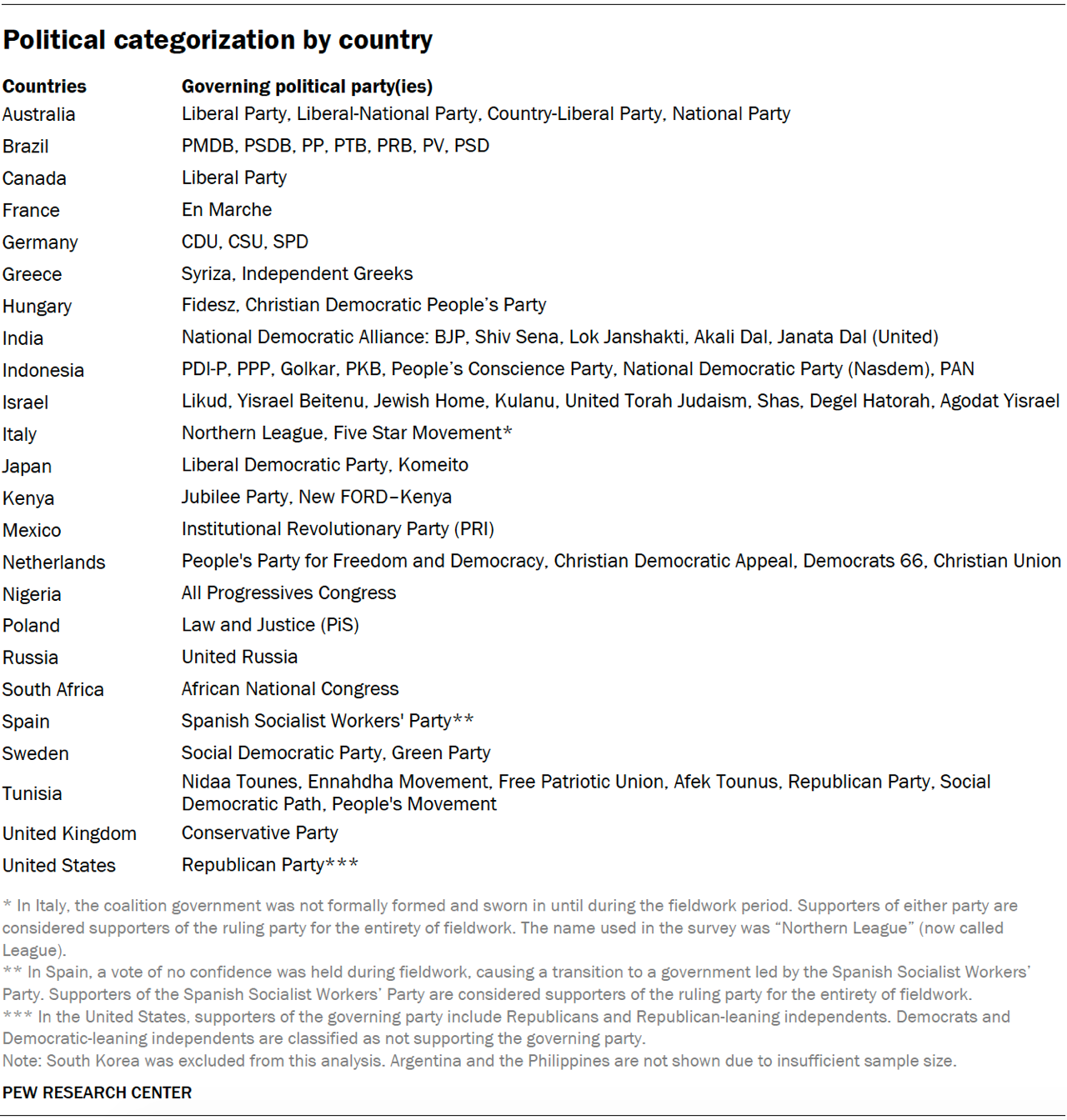This is a screenshot of an infographic by the Pew Research Center. In the bottom right corner, the Pew Research Center's name is displayed in a very small, capitalized black font. At the top of the infographic, a horizontal black line creates a boundary, mirrored by another black line at the bottom. 

Below the top line, aligned to the left, the title "Political Categorization by Country" is presented in bold black font. Directly beneath the title, there are two headings: "Countries" on the left and "Governing Political Parties" to the right. Both columns list their information vertically.

Under the "Countries" column, the first entry is "Australia," and under the corresponding "Governing Political Parties" column, the entries listed are "Liberal Party," "Liberal National Party," "Country Liberal Party," and "National Party." The next country listed is "Brazil," with the corresponding governing political parties "PMDB," "PSDB," "PP," "PTB," "PRB," "PV," and "PSD."

The infographic continues with Canada, which shows "Liberal Party" under its governing political parties. This pattern repeats for each country listed. The last entry is "United States," with the "Republican Party" listed under governing political parties, followed by three asterisks.

At the very bottom of the infographic, in light gray letters, there is an annotation explaining the meaning of the asterisks.